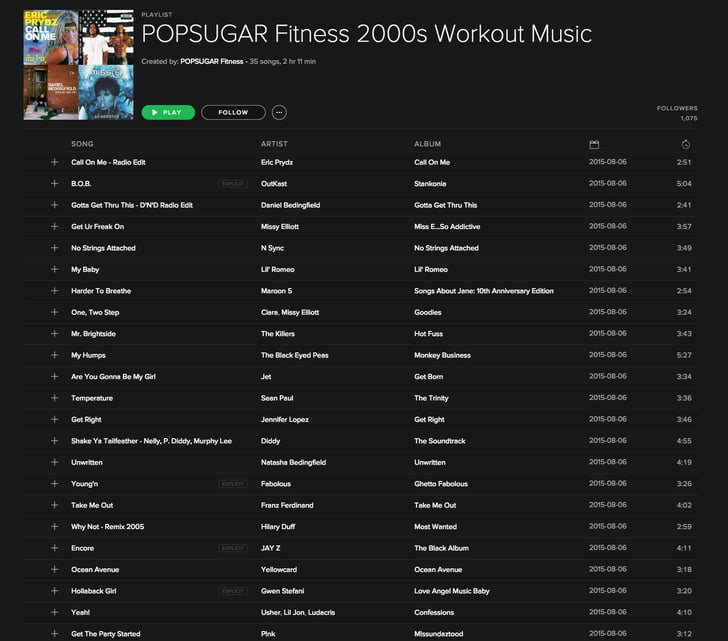The image features a Spotify playlist entitled "Sugar Pop Fitness 2000 Workout Music," curated by Sugar Pop Fitness. The playlist, located on the right side of the screen, is detailed in white text: "35 songs, 2 hours 11 minutes." At the top of this section, the word "Playlist" appears in smaller print.

In the background, the playlist showcases the first four album artworks. The first image appears to depict an 80s hair metal individual or possibly a woman with blonde hair in a tank top. The second image features the hip-hop duo OutKast standing in front of an American flag rendered as a mirror, showcasing two Black men. The third album cover, primarily red with white text, is not clearly identified. The fourth cover presents Missy Elliott, a Black woman with short black hair.

Beneath the playlist title, there is a green button with a white triangle labeled "Play." Adjacent to it is a white circle with black inner text that reads "Foul and White."

The playlist comprises songs that fit a high-energy workout vibe. Some notable tracks include:
- "Call On Me (Radio Edit)"
- "B.O.B"
- "Get Through This"
- "Get Ur Freak On"
- "No Strings Attached"
- "B.O.B (Baby)"
- "Harder to Breathe"
- "One, Two Step"
- "Mr. Brightside"
- "My Humps"
- "Are You Gonna Be My Girl"
- "Temperature"
- "Get Right"
- "Shake Ya Tailfeather"
- "Unwritten"
- "Youngin’"
- "Take Me Out"
- "Why Not"
- "Encore"
- "Ocean Avenue"
- "Hollaback Girl"
- "Yeah!"
- "Get the Party Started"